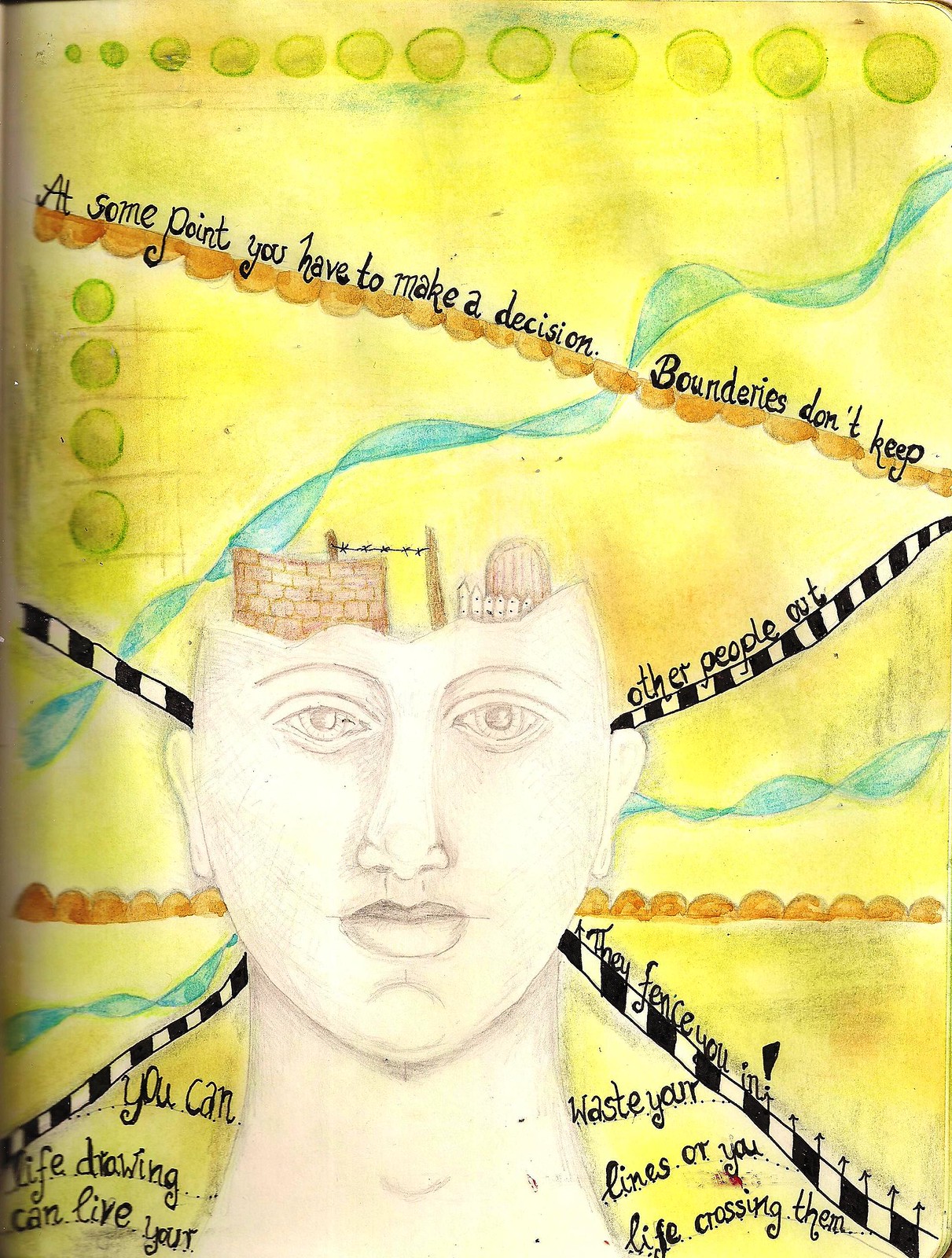The artwork features a yellow background, possibly painted or drawn in pencil, lending a handmade, artistic feel to the piece. The upper part of the image showcases a series of green circles that transition from smaller to larger as they move from left to right. Prominently, there's a detailed sketch of a person's head and neck, notable for its lack of hair and expressive facial features. The person’s eyes, nose, and large lips are clearly defined. Emanating from the head, there are multiple lines and ribbons, some resembling black and white striped ropes, giving a sense of dynamic movement or thought.

A brown, lacing pattern runs diagonally from the top left to the center, almost resembling a bridge, with the cursive text: "At some point you have to make a decision, boundaries don't keep." On the right side of the composition, additional text continues: "Other people out," emphasizing a narrative about boundaries. Further down, the artwork features the phrase: "You can waste your life drawing lines, or you can live your life crossing them," underscoring a rebellious or contemplative theme about life's constraints. Additional black and white striped lines, along with a blue ribbon, extend from the person's face towards the lower left corner, adding to the intricate and thought-provoking design.